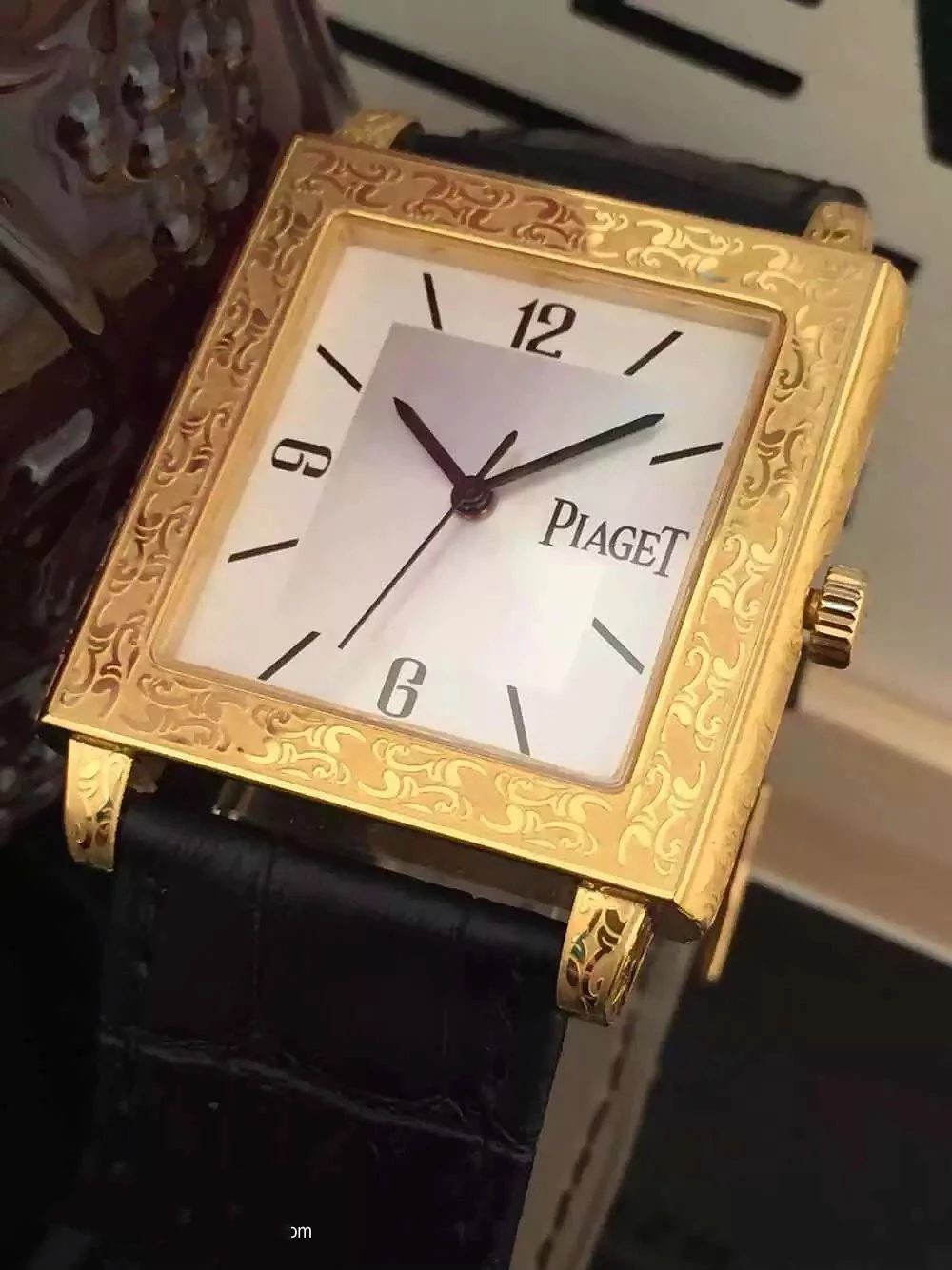This is a detailed, close-up color photograph of a luxury wristwatch by Piaget. The watch features a thick, gold square frame adorned with an intricate filigree and scrollwork design along the border. This design could either be decorative or possibly characters from another language, such as Arabic. The watch face itself is predominantly white with a central silver accent and black numerals. The numbers 12, 6, and 9 are marked clearly, while the other hours are indicated by thin, black diagonal dashes. The brand name "PIAGET" is prominently displayed where the 3 o'clock position would normally be. The watch has a small hand, a long hand, and a second hand, all of which are black. The time on the watch is set to approximately 10:10, with the second hand just before the 7. On the right side, there's a gold winding knob with indentations for grip. The watch is attached to a black alligator leather band, secured by two gold pegs at the top and bottom. The background of the image is simple, featuring black and white tones and possibly showing a baseboard along the bottom edge.